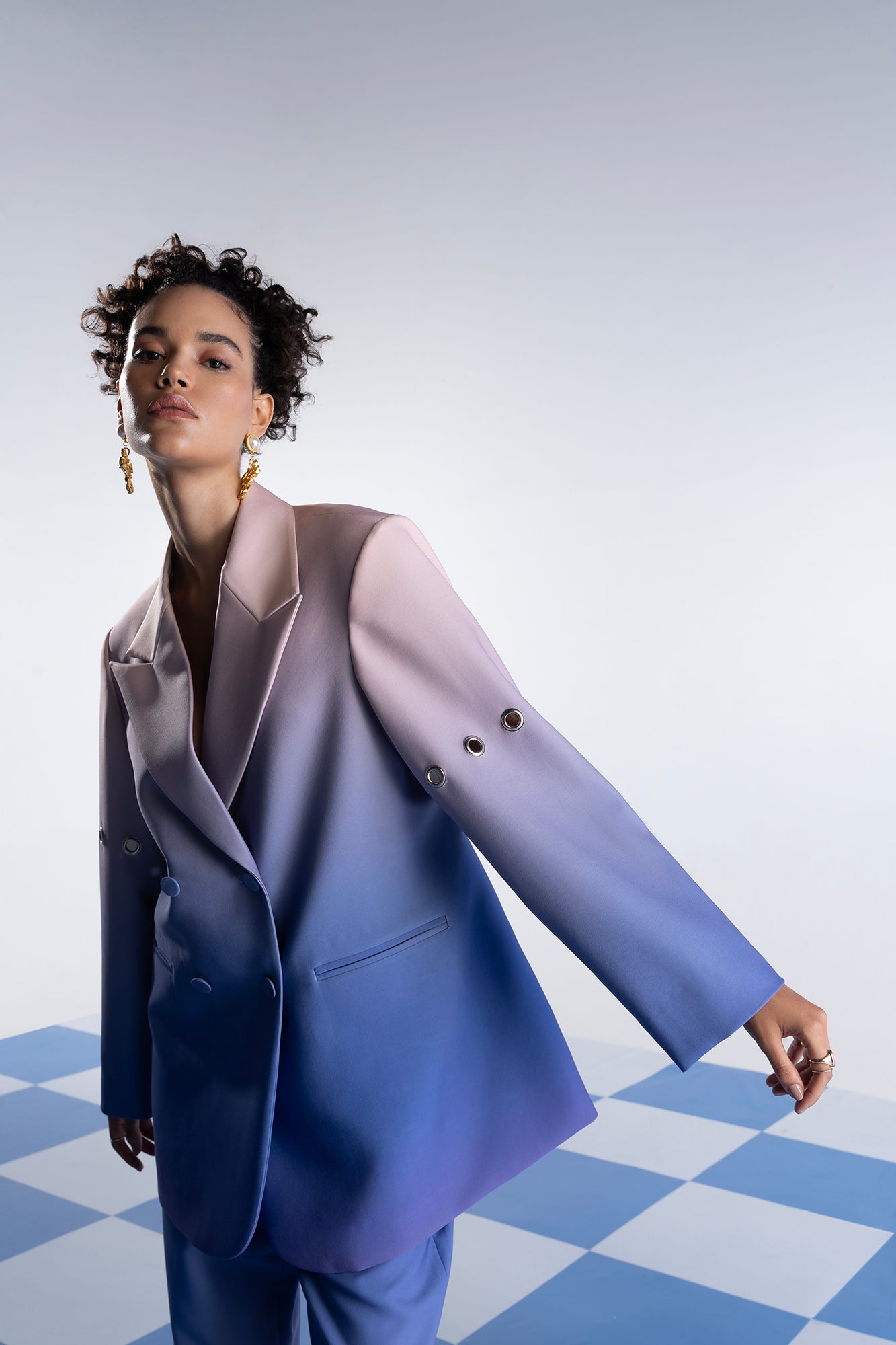The photograph features a young female model, approximately 20 years old, positioned towards the left side of the frame. She has short, tightly curled black hair and a very long, slender neck. Her light brown skin reflects a white light from the left side. She is dressed in a stylish power pantsuit with a double-breasted blazer that exhibits a striking pink-to-blue ombre gradient. The jacket is gray at the top and transitions through blue towards a light purple at the bottom. It features several cutout holes with gold grommets around the upper sleeves. The sleeves continue to a blue transition down to her hands, where her left arm is outstretched toward the right side at the bottom of the image. She wears large gold dangling earrings and a gold ring on her index finger.

Her expression is serious, and her head is turned back toward the viewer, creating a dynamic pose with her bent neck. The background consists of a gradient gray wall, transitioning from dark at the top to lighter at the bottom. The floor is a visually engaging checkerboard pattern of blue and white diamonds. The overall style is a blend of photographic representationalism, realism, product photography, and fashion photography, capturing the vibrant and detailed essence of the scene.